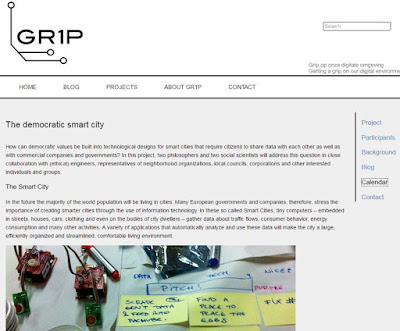The image is a screenshot taken from a website, distinctly divided into sections with various elements and text.

**Top Section:** 
- The top third features a plain white background.
- Below the white background, there is a black border that separates it from the rest of the content.

**Middle Section:**
- The remaining two-thirds of the image has a light gray background.
- In the top left corner, there is an outline of a black circle with a white interior.
- From this circle, a line extends downwards for about two inches before diagonally angling to the right for about an inch.
- At the bottom of this diagonal line, two horizontal lines stretch to the right for approximately an inch; one line is slightly above the other.
- At the end of the top horizontal line, there's a small circle.
- Large black lettering spells out "GR1P" prominently.
- On the right side, there is a small gray search bar with the word "search" within it, also in gray text.
- Beneath the search bar, there is a one-inch gap followed by the small, hard-to-read gray text "GRIPOP."
- Below this, black capitalized lettering spells out "HOME," "BLOG," "PROJECTS," "ABOUT," "GR1P," and "CONTACT," all separated by black lines that run horizontally across the width of the section.

**Bottom Section:**
- The light gray background begins prominently here.
- On the left side, the text "Democratic Smart City" introduces a paragraph spanned across four lines.
- Following a small space, the phrase "the Smart City" appears, leading into another five-line paragraph.
- The bottom of this section features an image showing scattered papers, with white papers on the left and yellow papers across the bottom right.
- In the top right corner of the gray section, there’s the word "PROJECT" in blue text.
- Underneath "PROJECT," the words "PARTICIPANTS in background," "BICG," a black-text word "CALENDAR" enclosed in a black outline, and "CONTACT" in blue text are listed consecutively.